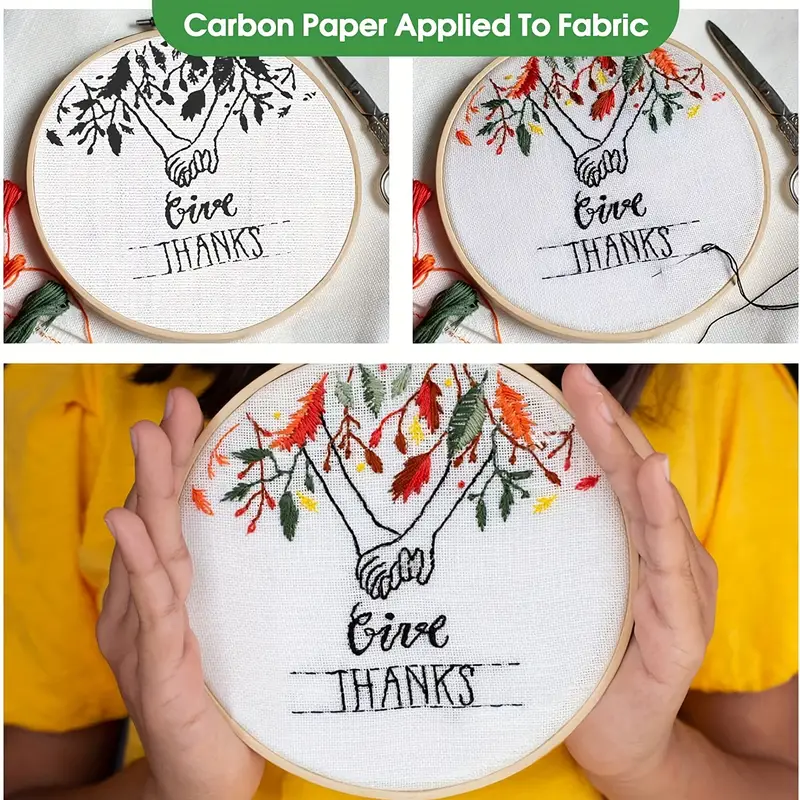This photograph showcases three stages of cross-stitching projects prominently displayed on white fabric backgrounds, all featuring the same design: two hands clasping each other beneath an array of leaves and above the words "Give Thanks." At the top, a green banner with white lettering reads "carbon paper applied to fabric." In the top left corner, the initial stage of the cross-stitching is shown within a light brown wooden frame, with black thread used to outline the hands, leaves, and text. The top right corner displays the same design, now completed with vibrant fall colors—orange, yellow, green, and red for the leaves. At the bottom, a woman in a bright yellow t-shirt proudly holds up the finished cross-stitch project, revealing a close-up view of the colored leaves in rich shades of red, orange, yellow, green, and dark red. Additionally, a pair of scissors can be spotted near the colored project on the right, adding a practical touch to the crafting scene. The photograph captures both the meticulous process and the rewarding final product of the cross-stitching endeavor.